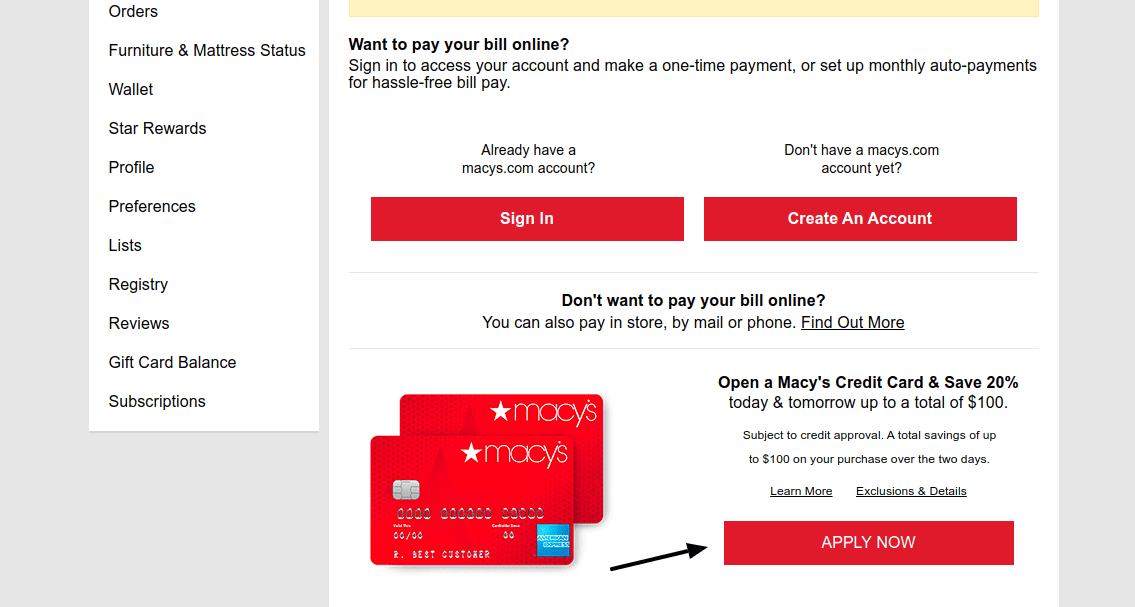On the left side of the image, a vertical white rectangle serves as a sectioned menu listing various links in separate rows: Orders, Furnace, Furniture and Mattress Status, Wallet, Store Rewards, Profile, Preferences, Lists, Registry, Reviews, Gift Card Balance, and Subscriptions. 

To the right, bold black text poses the question: "Want to pay your bill online?" Following this, it advises users to "Sign in to access your account and make a one-time or set up monthly auto payments for hassle-free bill pay." To the left of this, there's a prompt asking if a user already has a Macy's.com account, followed by an invitation to "Sign in." The words "Sign in" are enclosed in a red rectangle. Underneath, the text inquires: "Don't have a Macy's.com account yet?" with an option in red text to "Create an account."

At the bottom of the image, there are two red Macy's credit cards. Each features a white star beside the Macy's logo, spelled out as "M-A-C-Y-apostrophe-S." In the bottom right corner of each card, there's a blue box displaying the American Express logo. An arrow points to another red rectangle with the words "Apply Now." Above this, black text invites users to "Open a Macy's credit card and save 20%."